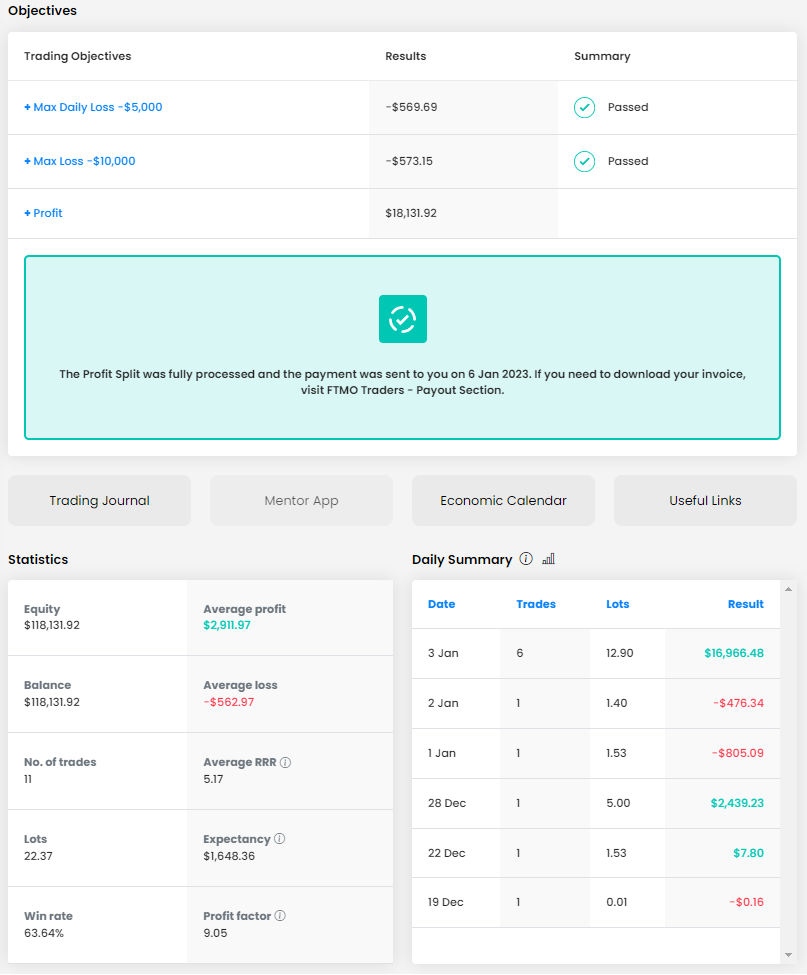Screenshot of a trading web page with a minimalistic design lacking a header.

At the top of the page, there is a thin gray border and a label on the left side that reads "Objectives." The background color is white, and the content consists of multiple charts and data elements related to trading activities.

The page is divided into three main columns at the top:
1. Trading Objectives
2. Results
3. Summary

Below these columns, three listings are displayed in a light blue font.

A very light green rectangle spans the full width of the page beneath the listings. Inside this rectangle, there is a slightly darker green square featuring a white check mark in the center, encircled by a pattern of white elongated dots. This section contains a message in black font that states: "The profit split was fully processed and the payment was sent to you on 6 January 2023. If you need to download your invoice via FTMOTraders payout section."

Further down, the page displays additional charts and data. There are four gray rectangles, each with a title:
- Trading Journal
- Mentor App
- Economics Calendar
- Useful Links

At the bottom of the page, the content is divided into two sections:
1. On the left, labeled "Statistics," featuring two columns of items.
2. On the right, labeled "Daily Summary," with four columns of data.